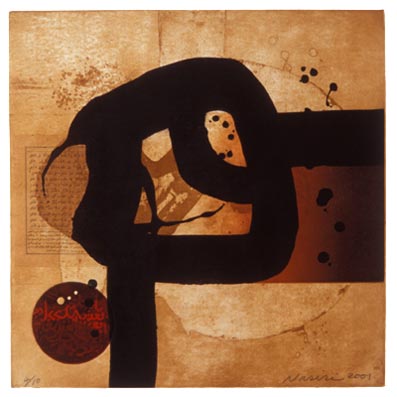The painting is an abstract piece on a light brown, tan-colored paper. Dominating the center is a black, serpentine shape that curves upwards and resembles an elongated, distorted letter "P." The form transitions into a horizontal strip that intersects with another vertical black stripe, creating an intricate, intertwined design. At the bottom left, there is a prominent red circle that evokes the image of a Christmas bulb, with black and white speckles inside it. Adjacent to this are scattered black paint splatter dots and a partially obscured red square adorned with additional black dots. The top left corner features a striking yellow patch complemented by touches of brown. Overlying the entire piece, faint and unreadable tiny text can be seen in the background towards the middle left section. In the lower right corner, an elusive artist's signature is present, with the year, possibly reading "2001" or "97," though it is difficult to decipher.